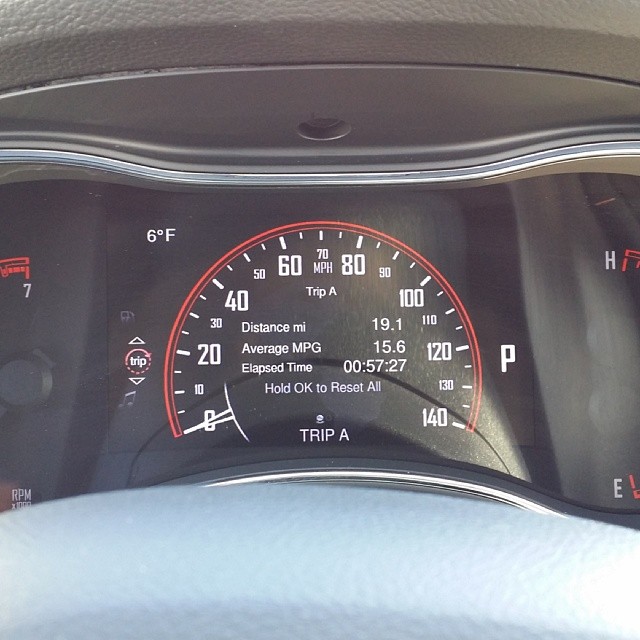The image captures a close-up view of a car's dashboard, revealing the speedometer and associated gauges. The central feature is the speedometer, which ranges from 0 to 140 and is bordered with a silver and red circular arc. The background of the dashboard is black, appearing to be covered with see-through plastic or glass. The numbers and details within the speedometer are predominantly white, providing clear contrast against the dark backdrop. 

The odometer displays 'Trip A' reading zero miles, with additional information noting '19.1 distance in miles,' '15.6 average miles per gallon,' and an 'elapsed time of 57 minutes and 27 seconds.' A prompt at the bottom of the speedometer indicates 'Hold OK to reset all.' To the left of the speedometer, there is a 'TRIP' button with up and down icons underneath it, and above this is a temperature gauge. The color palette of the dashboard features tan, black, silver, red, white, orange, and pink accents. 

The overall setting of the image appears to be outdoors during the day, viewed from just above the steering wheel with the interior of the car, including gray leather or faux leather sections, framing the bottom and sides of the photo. The elements and layout emphasize the clarity and functionality of the car’s dashboard instrumentation.